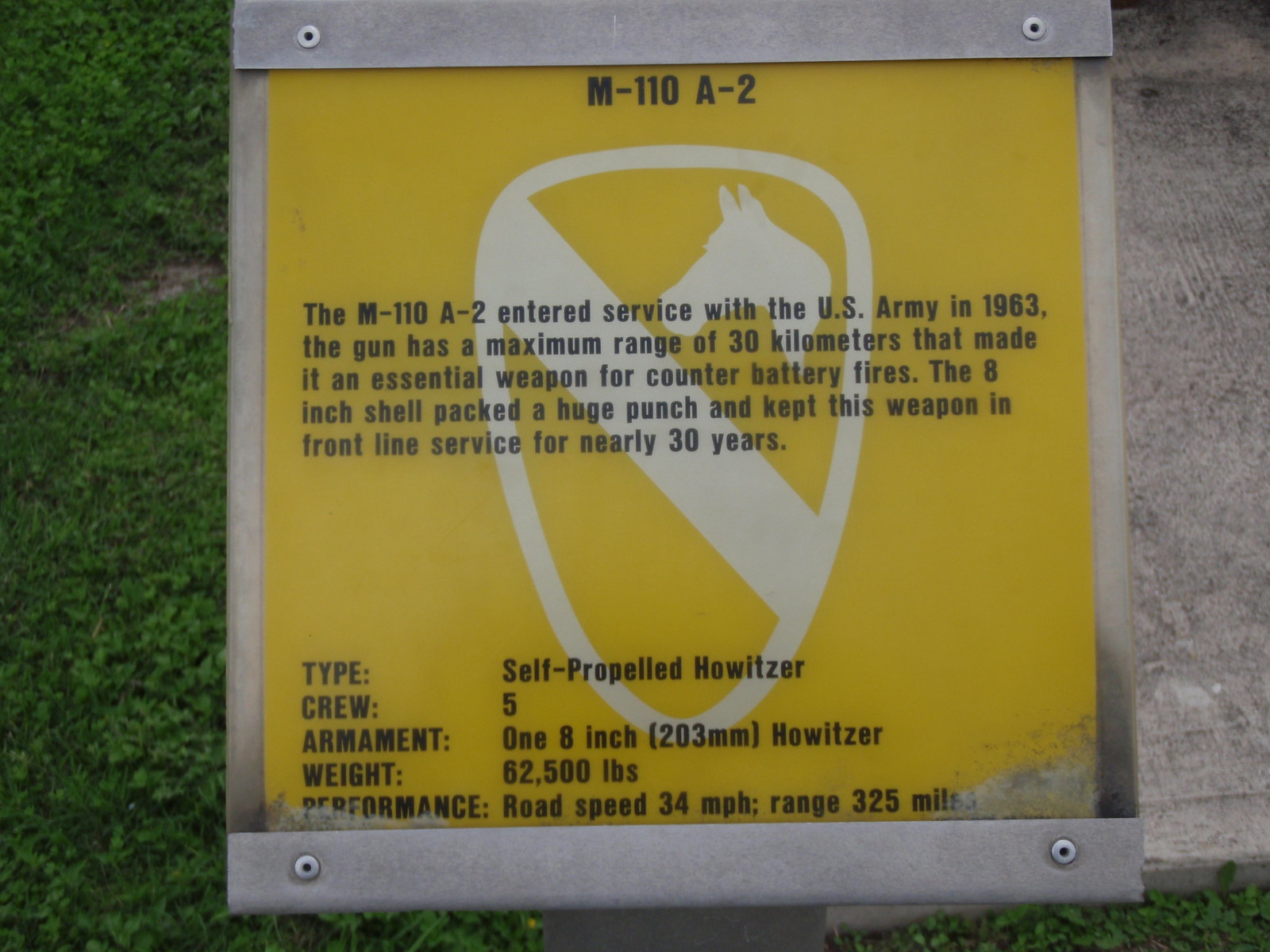This photograph, taken outdoors on a pre-overcast day, captures a yellow memorial sign framed in metal with rivets, set into a grassy area with some concrete and a cemented platform visible in the background. The sign's border is gray, and it features a central white oval crest with a diagonal stripe and a horse head in the upper right corner. The black text on the sign reads: "M-110-A-2." The detailed description continues: "The M-110-A-2 entered service with the U.S. Army in 1963. The gun has a maximum range of 30 kilometers that made it an essential weapon for counter battery fires. The eight-inch shell packed a huge punch and kept this weapon in front-line service for nearly 30 years." At the bottom of the sign, additional specifications are listed: "Type: Self-propelled howitzer. Crew: 5. Armament: 1 8-inch (203 millimeter) howitzer. Weight: 62,500 pounds. Performance: Road speed, 34 miles per hour. Range: 325 miles."